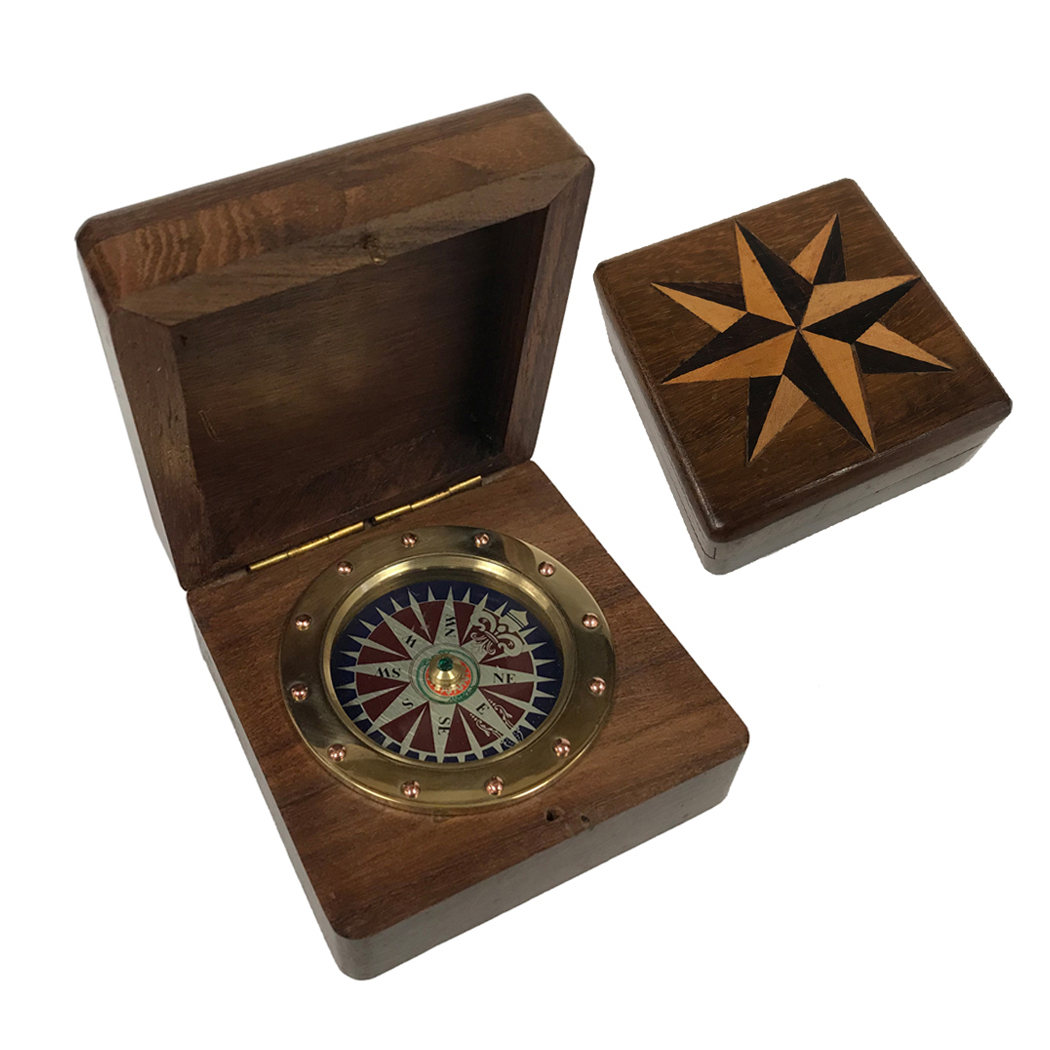The image features a meticulously crafted wooden box made of dark brown wood. This box contains a circular compass, which has a metallic gold border and intricate markings for various directions. The compass itself displays a combination of red, white, and blue colors. The box's lid, shown both open in the left side of the image and closed in the right, has a hinged design allowing it to cover the compass snugly. The lid's surface showcases a detailed star design made from contrasting light and dark brown woods, enhancing its elegant look. The entire setup is set against a solid white background, providing a stark contrast that highlights the deep hues and fine craftsmanship of the wooden box and its embedded compass.